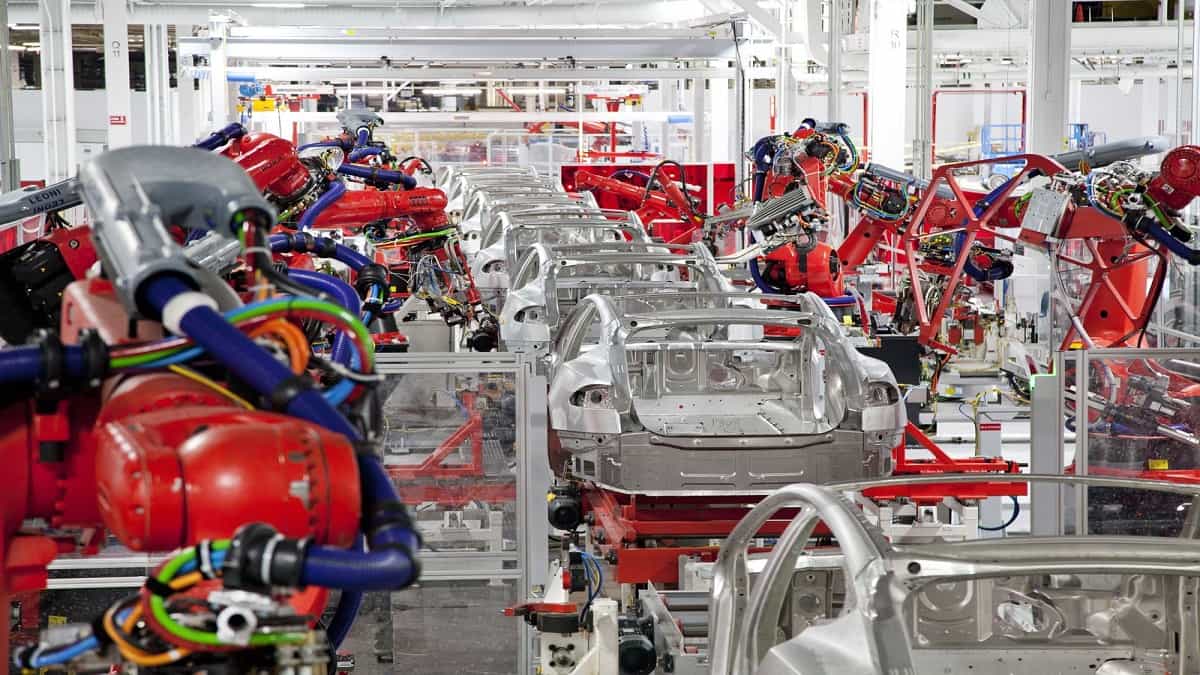This high-quality photo captures the bustling interior of an automobile manufacturing plant. Dominating the center is an assembly line featuring approximately seven to eight silver, unpainted car frames, each with a sporty coupe design characterized by a low, curved body. These skeletal car bodies, devoid of any features or equipment, move along the line, elevated on a mechanized conveyor system.

Flanking both sides of the assembly line are numerous robotic arms, predominantly red, equipped with a network of brightly colored tubing in hues of blue, yellow, green, and orange. These robotic arms diligently work on assembling various parts onto the car frames. The factory floor, made of concrete with a silvery hue, is meticulously organized, reflecting a high degree of precision and coordination.

The walls and ceiling of the factory are a clean, stark white, creating a bright and well-lit environment that contrasts sharply with the vivid colors of the machinery. The entire scene is framed by steel structures, reinforcing the industrial ambiance of the facility. This photograph eloquently captures the intricate and efficient process of modern car manufacturing.